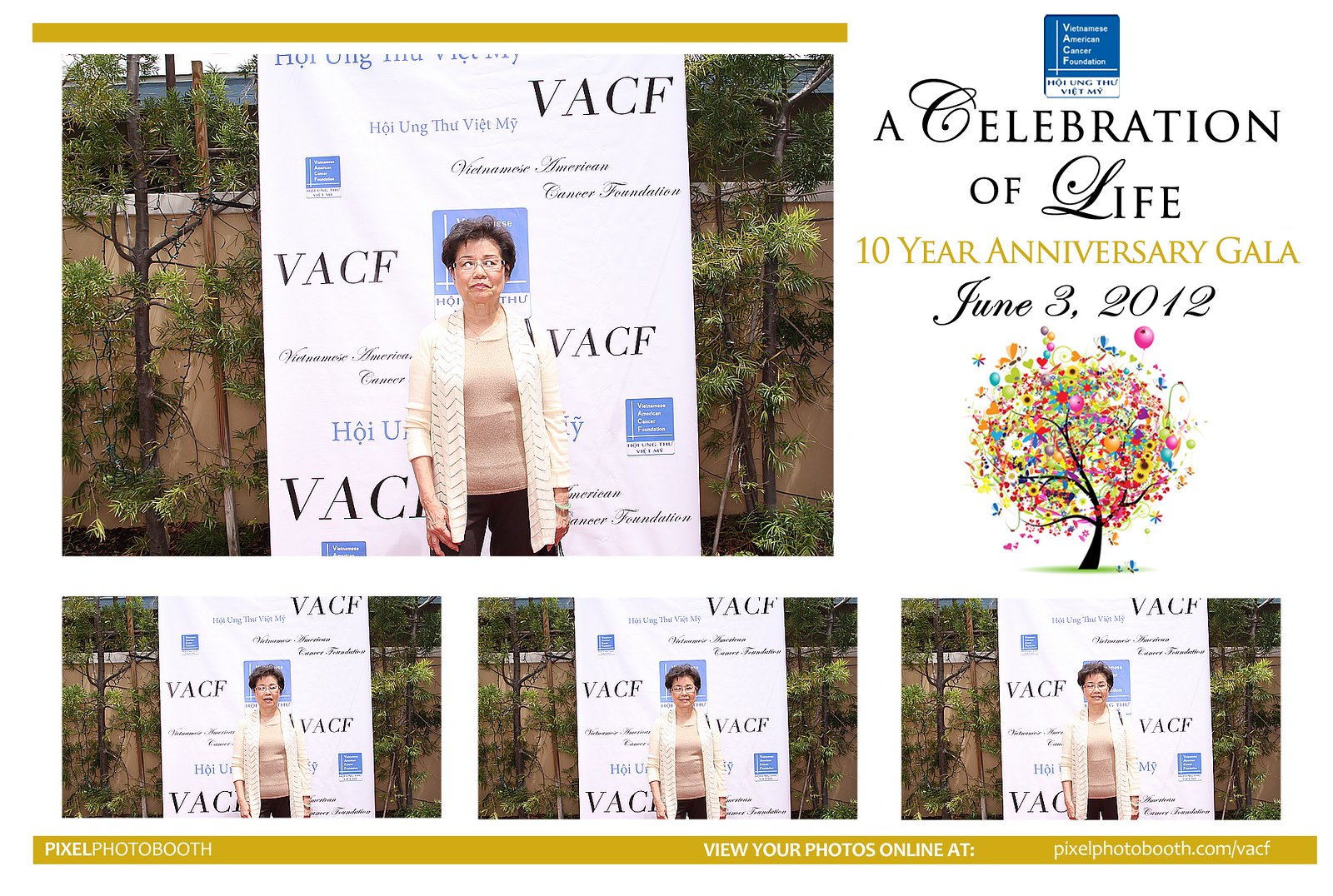This image is a collage of four photographs featuring an Asian woman with short black hair, glasses, and dark eyebrows, standing in front of an event banner. She is wearing a beige cardigan over a cream shirt, brown pants, and a jade bracelet on her left hand. The banner behind her reads "VACF, Vietnamese American Cancer Foundation," and is positioned outdoors with trees and leaves visible in the background. The banner signifies a "Celebration of Life, 10-Year Anniversary Gala" held on June 3rd, 2012. Additionally, there is a colorful, whimsical illustration of a tree composed of balloons, butterflies, and flowers on the banner. The woman, who appears serious and is not smiling, is seen in one large image and three smaller duplicates underneath.